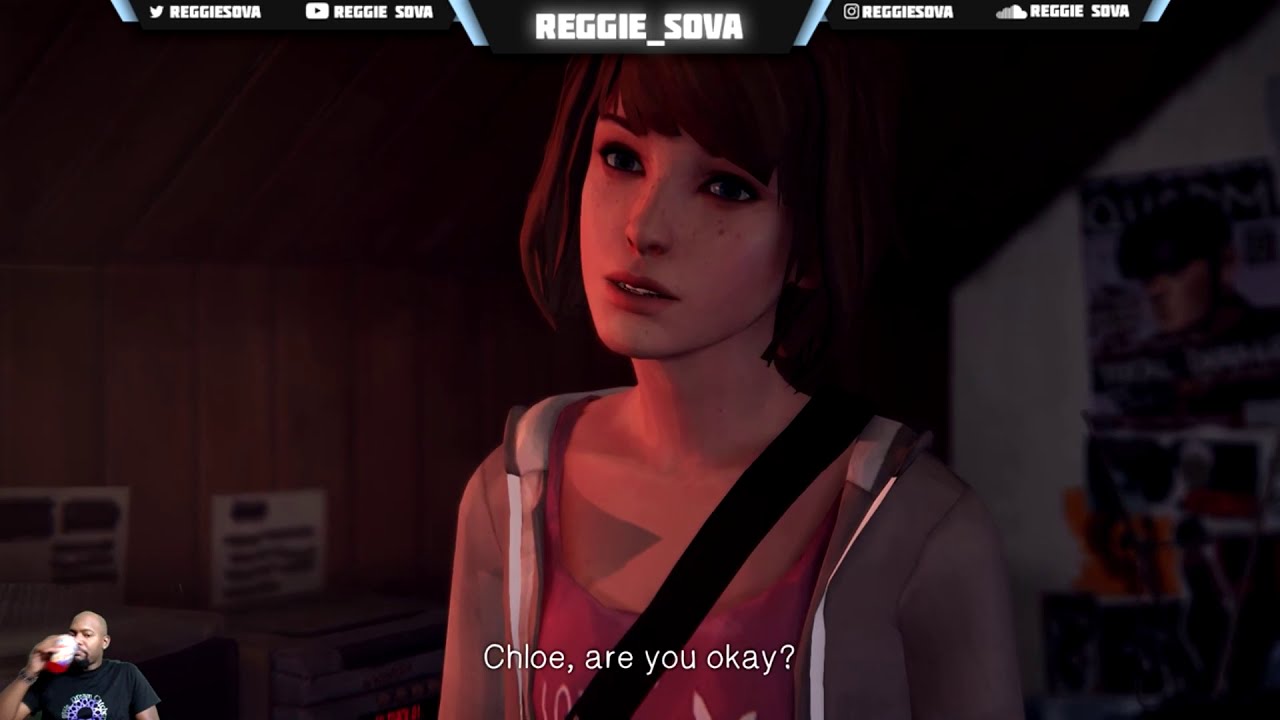The image is a screen capture from a video game featuring a close-up of an animated young girl with red-brown, short hair and freckles. She is wearing a zip-up hoodie and a pink t-shirt underneath, with a black strap across her chest suggesting she is carrying a backpack or bag. The background shows a brown paneled wall, and there is a poster resembling a magazine on the right side. On the screen, white text reads, "Chloe, are you okay?" superimposed in front of the character. At the top of the image, there is text that says "Reggie_Sova" along with icons for Twitter, YouTube, Instagram, and SoundCloud, indicating this is being streamed by a user named Reggie Sova. In the lower left corner, there is an inset image of the streamer, a bald black man with a goatee, wearing a black t-shirt and in the act of drinking from a cup.